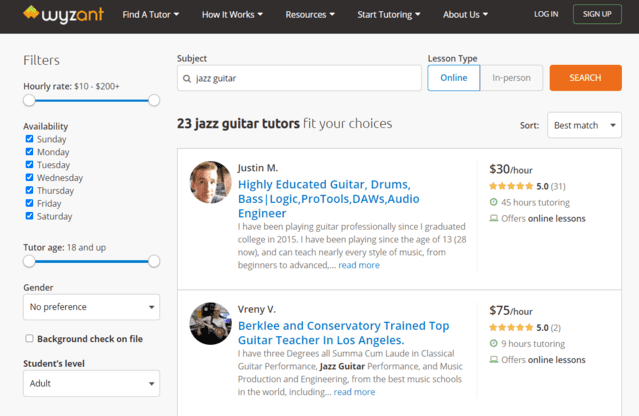The image is a screenshot from the WYZANT website. At the top, there is a brown bar stretching horizontally across the upper portion of the screen. On the left side of this bar, there is a white font horizontal menu with several options: "Find Your Tutor," "How it Works," "Resources," "Start Tutoring," and "About Us." On the far right of the brown bar, there are two buttons: "Log In" and "Sign Up."

On the left-hand side of the screen, a vertical menu serves as a filter panel. The panel heading, "Filters," is displayed in large black font. The first filter option, "Hourly Rate," features a slider bar allowing selection from $10 to $200 plus. Below this, the "Availability" section lists each day of the week vertically with checkboxes, all of which are checked. The next filter option is "Tutor Age," starting from 18 and up. Following this is the "Gender" filter option, a checkbox for "Background Check on File," and finally, the "Student Level" filter where the selection “Adult” is chosen.

To the right of the filter panel, it displays a summary: "23 Jazz Guitar Tutors," indicating the number of tutors available based on the selected filters.